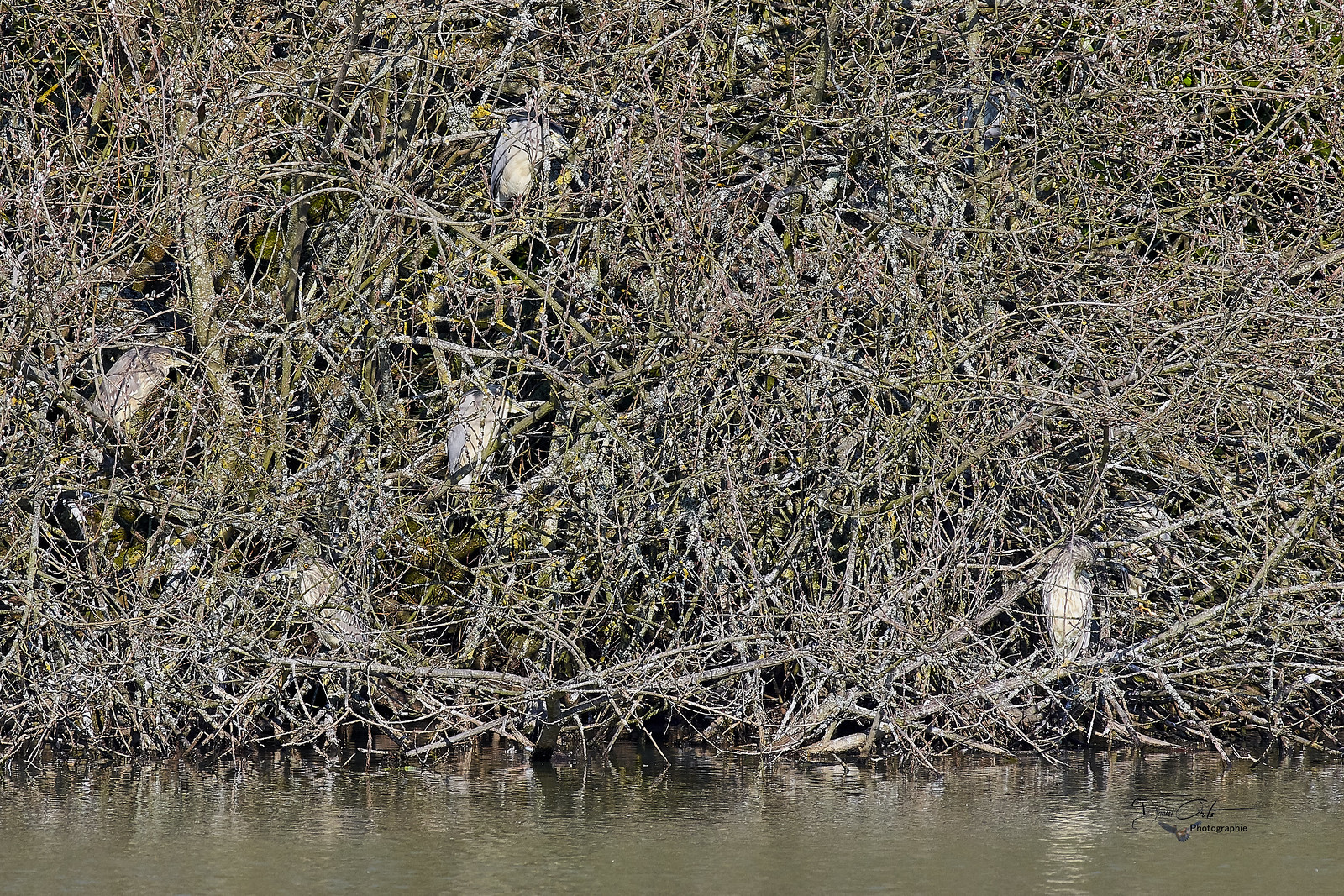The image depicts a serene yet murky shoreline, likely along a swamp or riverbank, characterized by calm, greenish-brown waters. The shore is densely covered with tangled branches, tall grasses, and various undergrowth, giving an impression of a rugged, natural area. Amidst this wild brush, five grayish-white birds are subtly camouflaged. At first glance, the birds might blend seamlessly with their surroundings due to their muted colors and the chaos of branches. On closer inspection, one can make out their distinctive features: whitish-gray plumage, long white beaks, and small, black eyes. Four of them appear to be facing away or in a side profile, emphasizing their ability to blend into the environment, while one bird’s beak is more prominent, providing a slight hint of their presence amid the tangled shore vegetation.